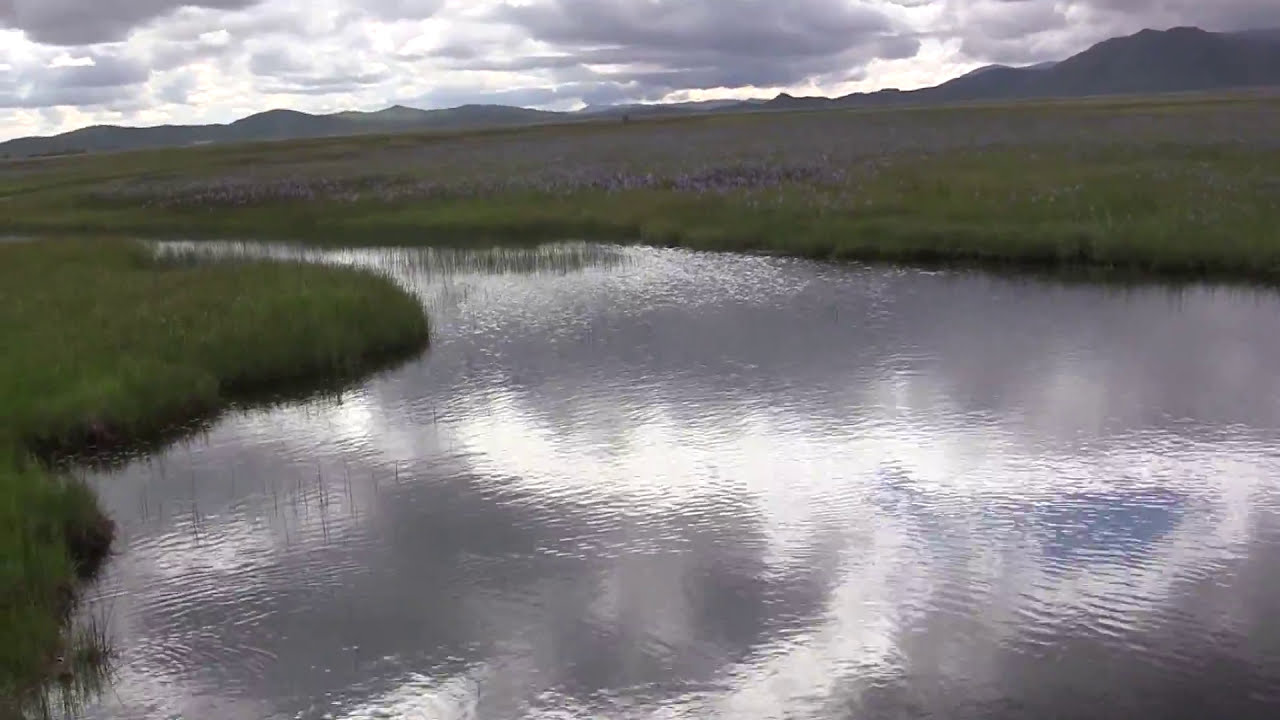In the serene scene depicted, a reflective lake captures the moody overcast sky, punctuated by occasional patches of blue and sunlight breaking through the thick clouds. Surrounding the water are lush patches of tall, green grass, giving way to a field dotted with purple and white wildflowers, likely lavender. The landscape extends to rolling hills and towering mountains that frame the background, their dark green hue softened by the distance. The wetland scenery showcases a stream flowing into the lake from the left, enhancing the natural beauty of this national park. The sky, filled with large fluffy clouds, adds a dramatic contrast to the tranquil water below, highlighting the harmonious blend of land, water, and sky in this picturesque outdoor setting.